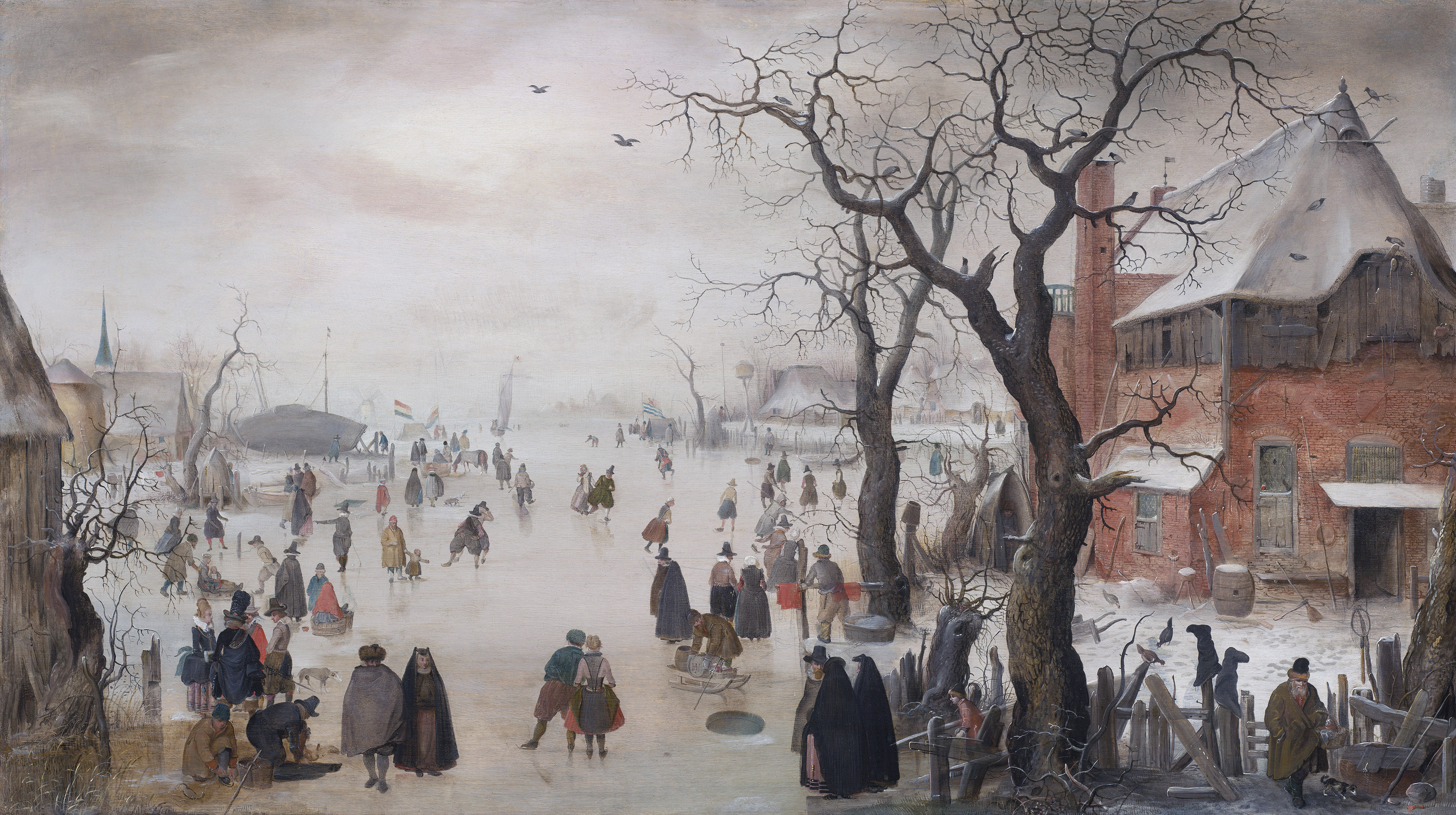This image captures a bustling winter scene that appears to take place around the mid-1800s, possibly in a small French village during a gray, snowy day. The centerpiece of the image is a frozen lake, used as an ice skating rink, where around 30 people are either skating with children or standing and watching. The attire of the people suggests a historical setting reminiscent of the Salem Witch Trials era, enhanced by the presence of two nuns in the foreground.

To the right, a dilapidated brick building stands prominently with its white, snow-covered arched roof. This four- to five-story structure features broken glass and weathered wood paneling. Adjacent to this building, a rugged wooden fence, on top of which boots are hung to dry, encircles a large, barren tree. A man in a brown coat is seen near this fence, adding to the scene's historical ambiance. Nearby, a barrel rests against the building, and two large trees stand prominently beside it.

In the background, more trees, similarly leafless, line the edge of the frozen lake. On the left side of the image, we can see the corner of a granite building and another structure in the distance, along with a flag that appears to be French. In the far distance, there’s a steeple, possibly of a church, adding to the village feel. The sky is a mix of dark gray and white, typical of a wintry atmosphere, with two birds flying overhead. All these details blend to depict a vibrant, yet somber winter day in this historical village.